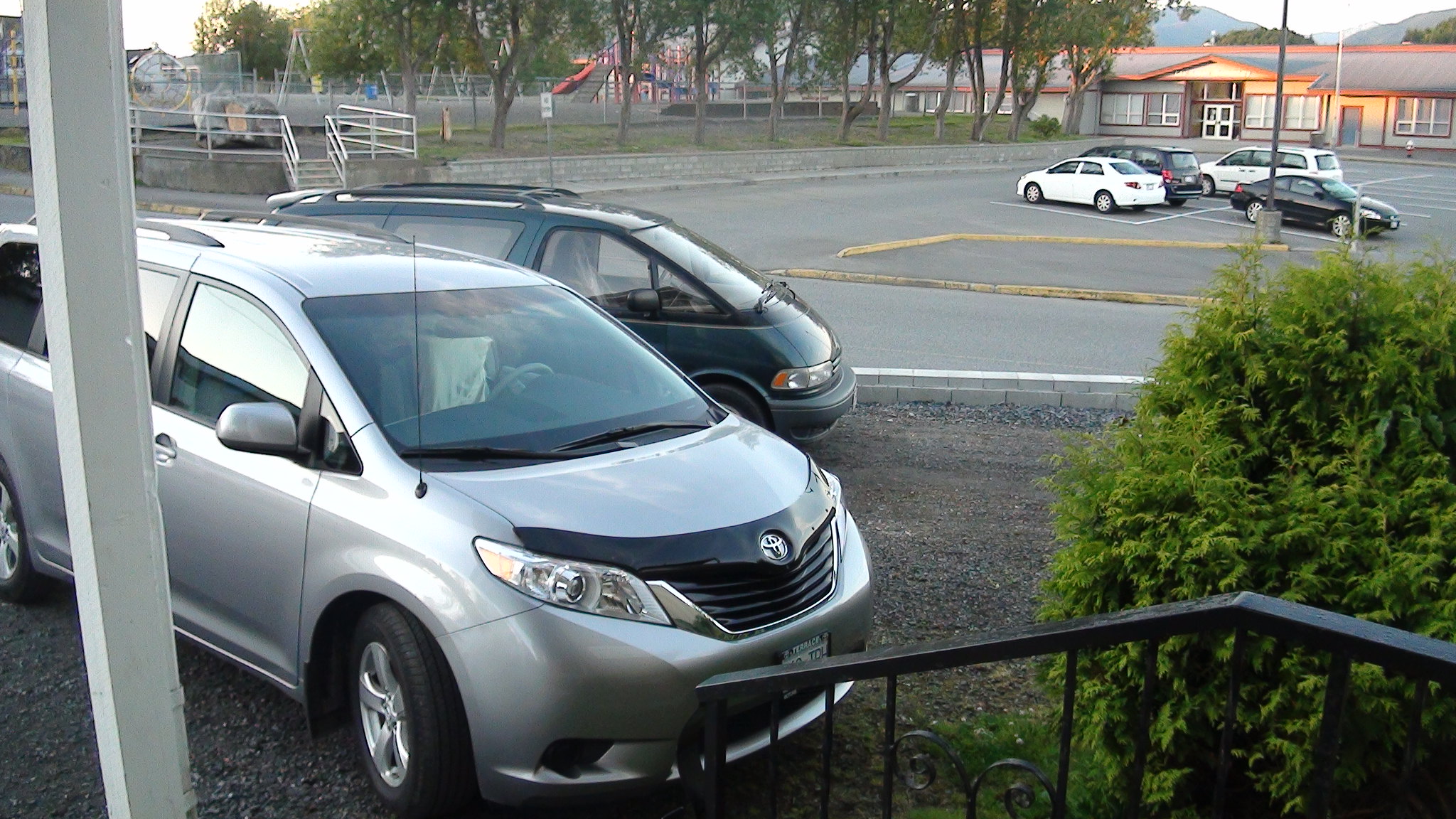This daytime photo, likely taken from a front porch or office entrance, captures an exterior scene featuring a parking area. In the foreground, a black wrought iron railing and a white wooden post mark the steps leading up to a presumed house. Adjacent to the railing, a lush green bush adorns the scene, while the ground nearby consists of gravel and dirt. Two minivans—one a silver Honda and the other a dark green older model—are parked in this space, instead of using the parking lots in the background.

Behind the minivans, there's a larger parking lot filled with various cars, mainly white and black, which belongs to a substantial, single-floor building that appears to be a school. This building, light brown with clay-colored siding and white doors, stretches across the image, suggesting it can accommodate many people. On the left-hand side of the parking lot, there's a playground with amenities like tire swings and a playset. Towering trees provide a backdrop to this area, enhancing the overall sense of a community-focused educational environment.